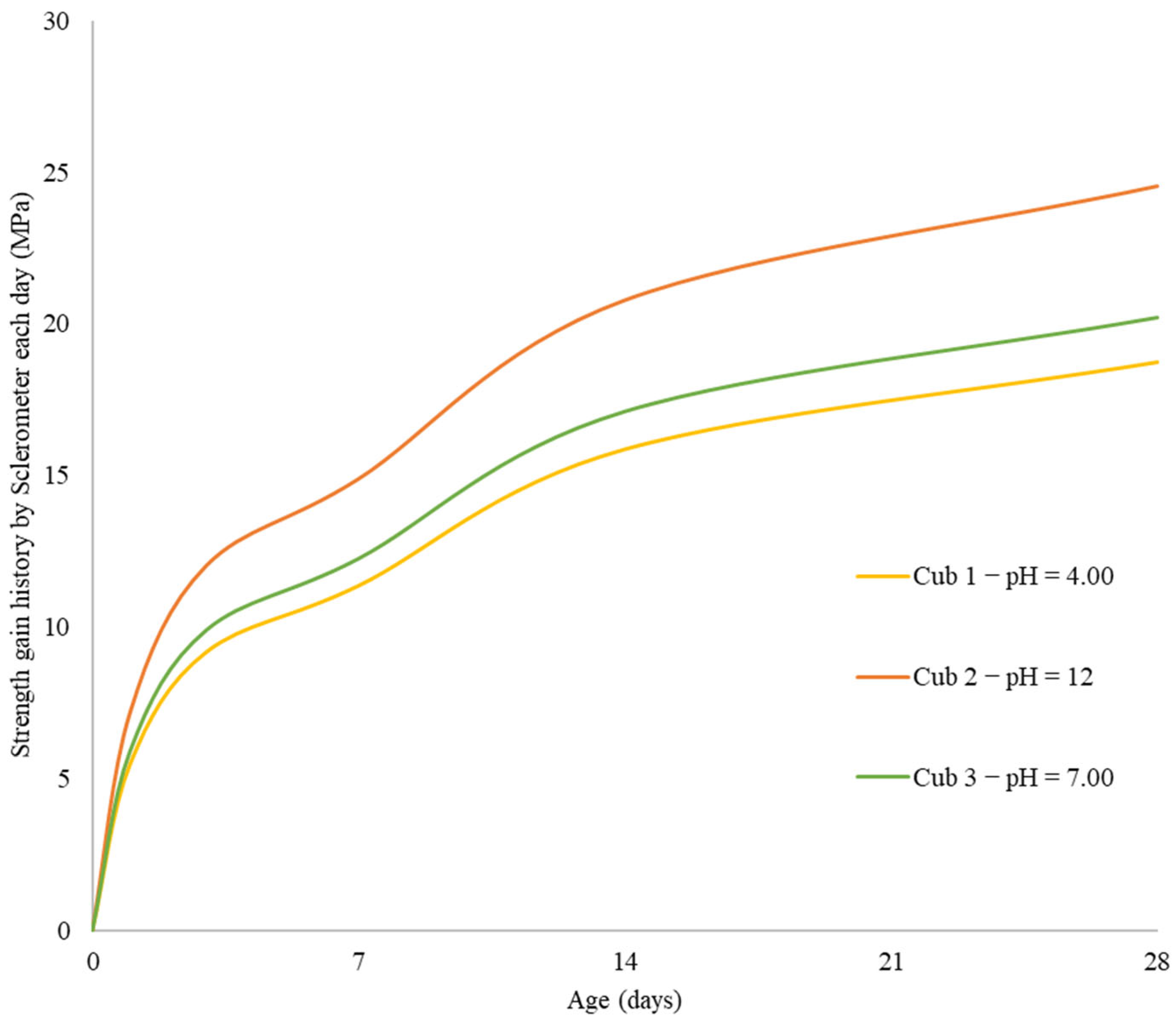This image depicts a detailed scientific chart illustrating strength gain history measured by a sclerometer each day, with results expressed in megapascals (MPa). The vertical y-axis ranges from 0 to 30 and is labeled "Strength Gain History by Sclerometer Each Day (MPa)." The horizontal x-axis spans from 0 to 28 days, marked with increments at 0, 7, 14, 21, and 28 days, and is labeled "Age (days)." 

The chart features three color-coded lines representing different samples with varying pH levels. The red line, labeled "cub 2, pH 12," demonstrates the highest strength gain over time. The green line, labeled "cub 3, pH 7," follows in performance, showing a moderate strength gain. Finally, the yellow line, labeled "cub 1, pH 4," shows the lowest strength gain.

All three lines indicate an initial rapid increase in strength gain, which decelerates into a more gradual incline. The chart provides a clear comparative analysis of how pH levels affect the rate of strength gain in the samples over a 28-day period, with cub 2 consistently outperforming the other samples.